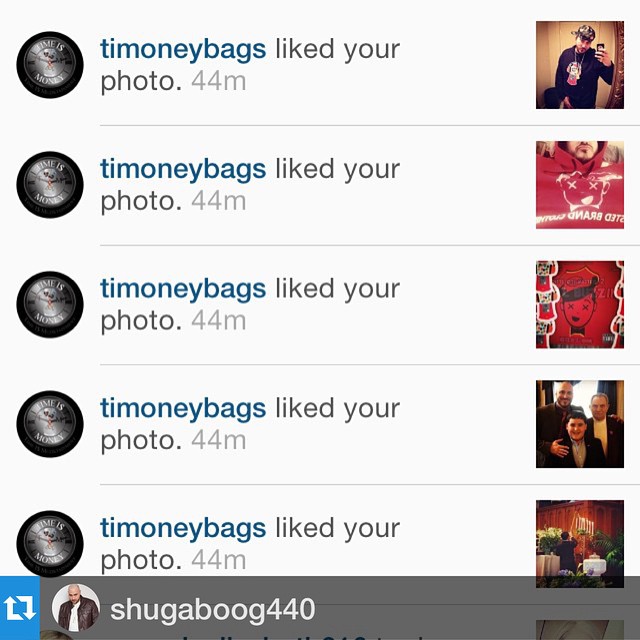This image is a screenshot of social media notifications showing one user's activity. It consists of five sections, each starting with "Timoni Moneybags liked your photo" in blue text, with "44M" indicating the time of each action. To the left of this text is a black circle with a gray center, likely Timoni Moneybags' profile picture. On the right side of each section, there is a corresponding photo that received the like. 

The first photo features a man holding up a phone, taking a selfie while wearing a black shirt. The second is a close-up shot of a man's chest, visibly wearing a red shirt with white lettering, shown from the nose down. The third photo stands out with its red background and the black silhouette of a face, with black hair, eyes, and mouth. The fourth image includes three people: a tall man on the left, a child in the center, and another man on the right, resembling a family portrait. The fifth and final picture shows a person lighting candles on a menorah, hinting at a celebration, possibly during Hanukkah.

Below these sections is a gray bar spanning the width of the image. On the left side of this bar, there is a blue square featuring up and down arrows. Next to this, in the gray bar, is a circular profile picture of a bald-headed man in a brown coat and white shirt, followed by the text "Sugar Boog 440," indicating the account receiving the likes.